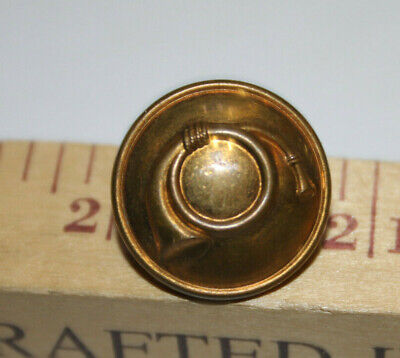This is an image of a small, vintage brass or bronze military coat button, prominently featuring a detailed bugle design in its center. The button is circular and shows signs of age with a slight discoloration. It rests on a wooden ruler with red markings, positioned to indicate its size, which appears to be around half an inch in diameter. The ruler is marked with partly visible letters 'R-A-F-T-E-D' and displays measurements from the two to two and a half-inch marks. The background of the image is light gray, further emphasizing the antique appearance of the button and the aged feel of the ruler.